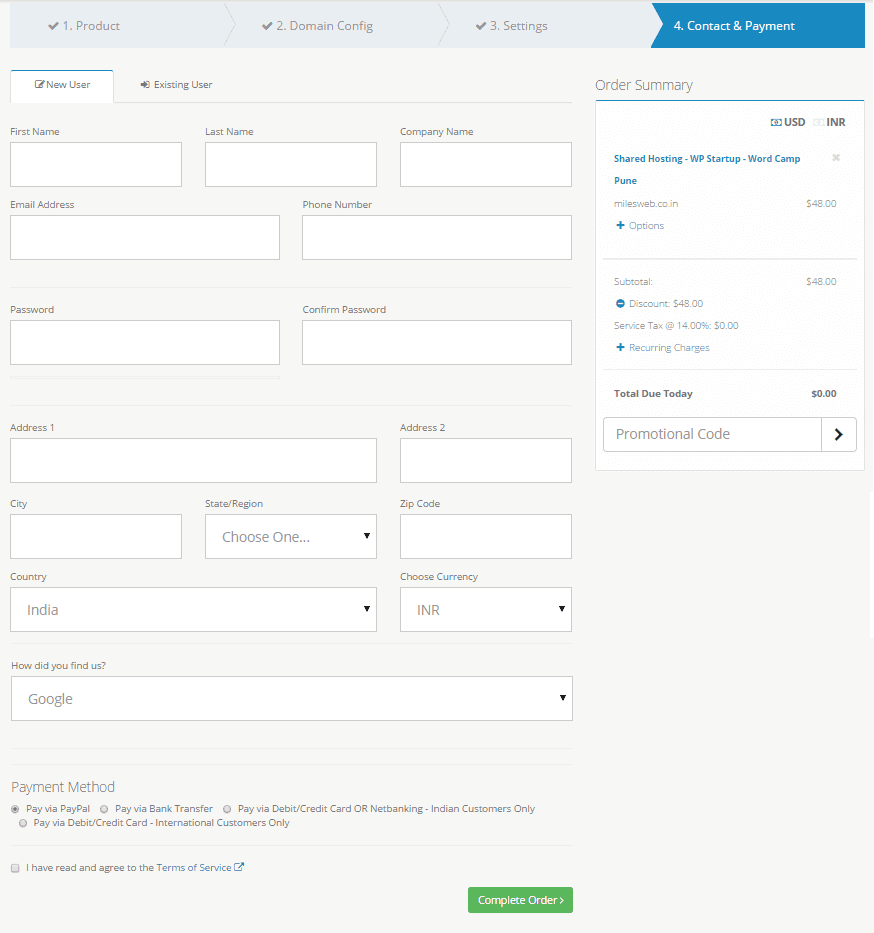The image depicts a detailed contact and payments page, specifically an order summary section, of a web form. The interface suggests that the user has progressed through various sections – including products, domain configuration, and settings – and has now reached the "Contact and Payments" step, as indicated at the top right of the page.

Just below this header, a notice states "New User." The form begins with a series of mini text entry boxes for personal information: "First Name," "Last Name," and "Company Name." The subsequent line includes entries for "Email Address," "Phone Number," "Password," and "Confirm Password." 

Further down, the form asks for address details: "Address Line 1" and "Address Line 2," followed by text entry fields for "City" and a drop-down box for selecting the "State." After that, a field for "Zip Code" is provided. 

The form then prompts for "Country," which is displayed as a drop-down menu currently set to "India." The next field is for "Choose Currency," defaulted to "INR," the Indian currency. The last piece of contact information requested is "How Did You Find Us?" which shows "Google" in the text box.

At the bottom of the form, smaller text lists the various payment methods available. Finally, a prominent green “Complete Order” button serves as the call-to-action for finalizing the form submission.